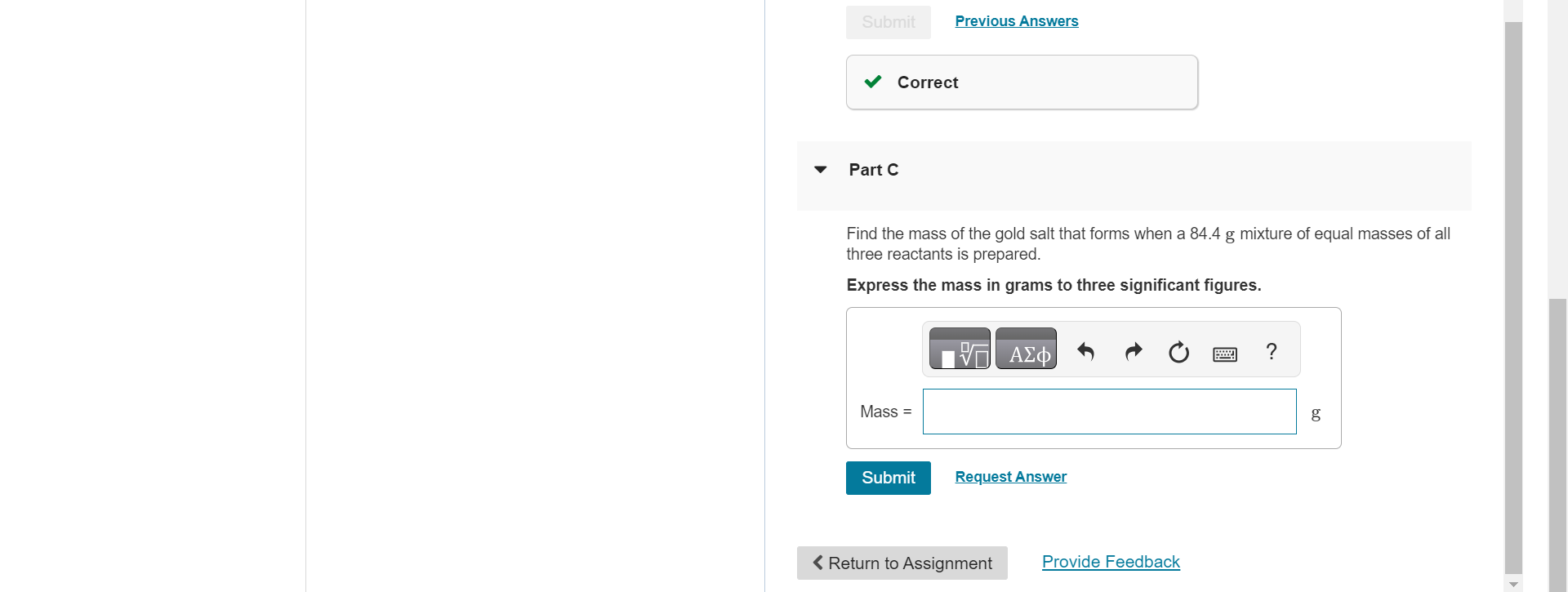### Detailed Caption for the Image

The image shows an online interface mostly featuring a white background with some informational and functional elements.

At the top of the interface, there's a gray text labeled "Submit" and a blue text labeled "Previous Answers." Below this, there is a box containing a green check mark accompanied by the word "Correct" in black font.

Further down, there is a dropdown arrow labeled "Part C," followed by a text instructing the user: "Find the mass of the gold salt that forms when an 84.4 g mixture of equal masses of all three reactants is prepared." This is followed by a prompt in bold black text: "Express the mass in grams to three significant figures."

Below this text, there are several icons:
- A division icon represented as a couple of different squares
- An A sigma omega button
- A reply button depicted as an arrow pointing to the left
- A forward button depicted as an arrow pointing to the right
- A refresh button depicted as a circular arrow
- A keyboard icon
- A question mark icon

Underneath this row of icons, there is a text input field labeled "Math equals," with a box for entering numerical values (labeled "G"). There are also two buttons: one labeled "Submit" and another option labeled "Request Answer."

At the bottom of the interface, there are links to "Return to Assignment" and "Provide Feedback."